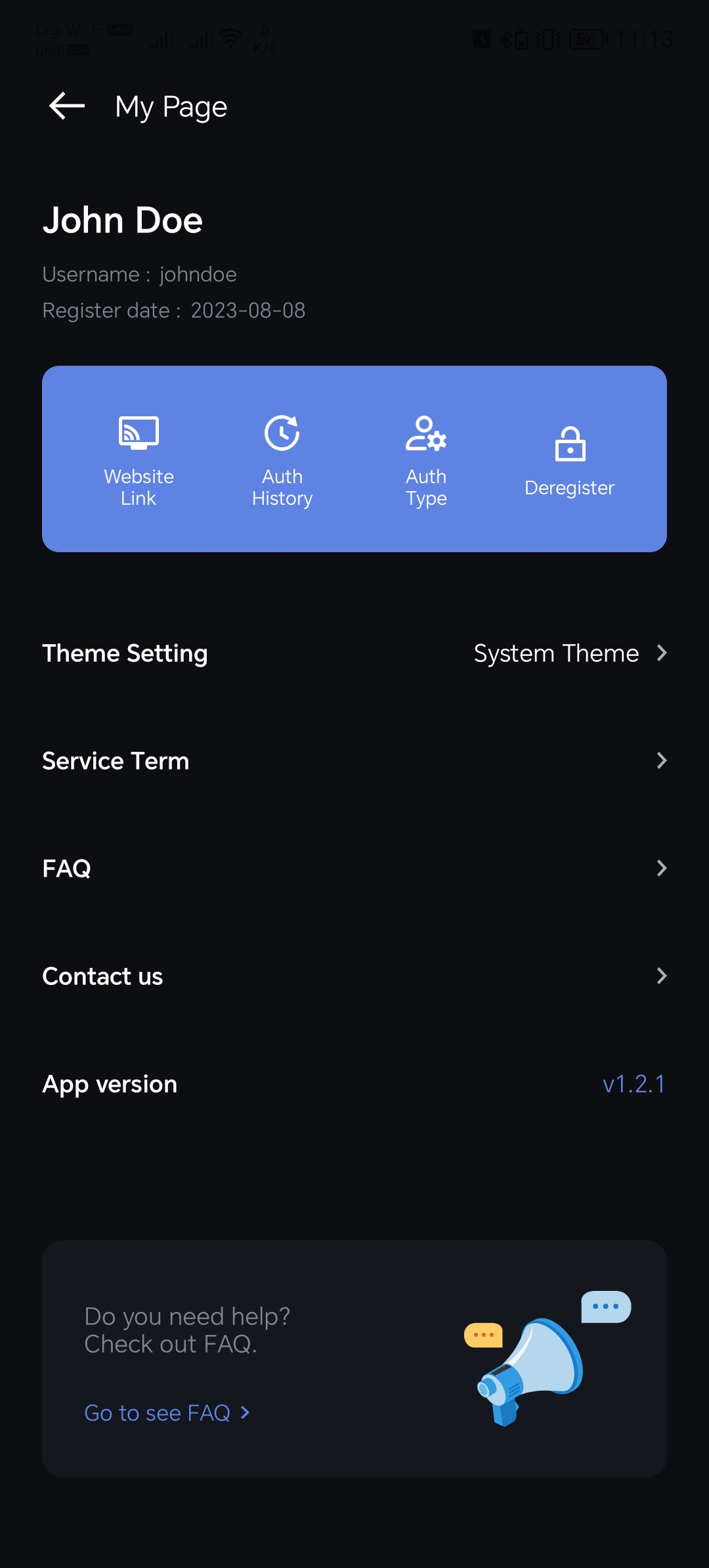The top section of the image features a white arrow pointing left, accompanied by the text "My Page." Directly below, the name "John Doe" appears in white text. There are two lines of very small gray text beneath this name, containing information that includes the register date and the date "2023 08 08," though the text is quite difficult to read.

Moving further down, there is a blue rectangle. Inside this rectangle, on the left, the text "Website Link" is present, alongside an image resembling a computer screen. Above this, the label "AUTH History" is displayed. Adjacent to this, a circular image is positioned above the term "AUTH Type," finally indicating the status "Unregistered" beside an image of a small square with a dot inside, written in very small text.

Below this section, aligned to the left, the text "Theme Setting" is displayed in white. About four inches to the right, the text "System Theme" appears with a small arrow pointing to the right. Beneath this, the label "Service Term" is shown, followed by a right-pointing arrow, and then "FAQ" in all capital white letters. Continuing downward, "Contact Us" is tagged along with "App Version." At the very bottom of the image, the text reads "Do you need help? Check out FAQ," complemented by a blue speaker icon emitting a speech bubble containing three small dots.